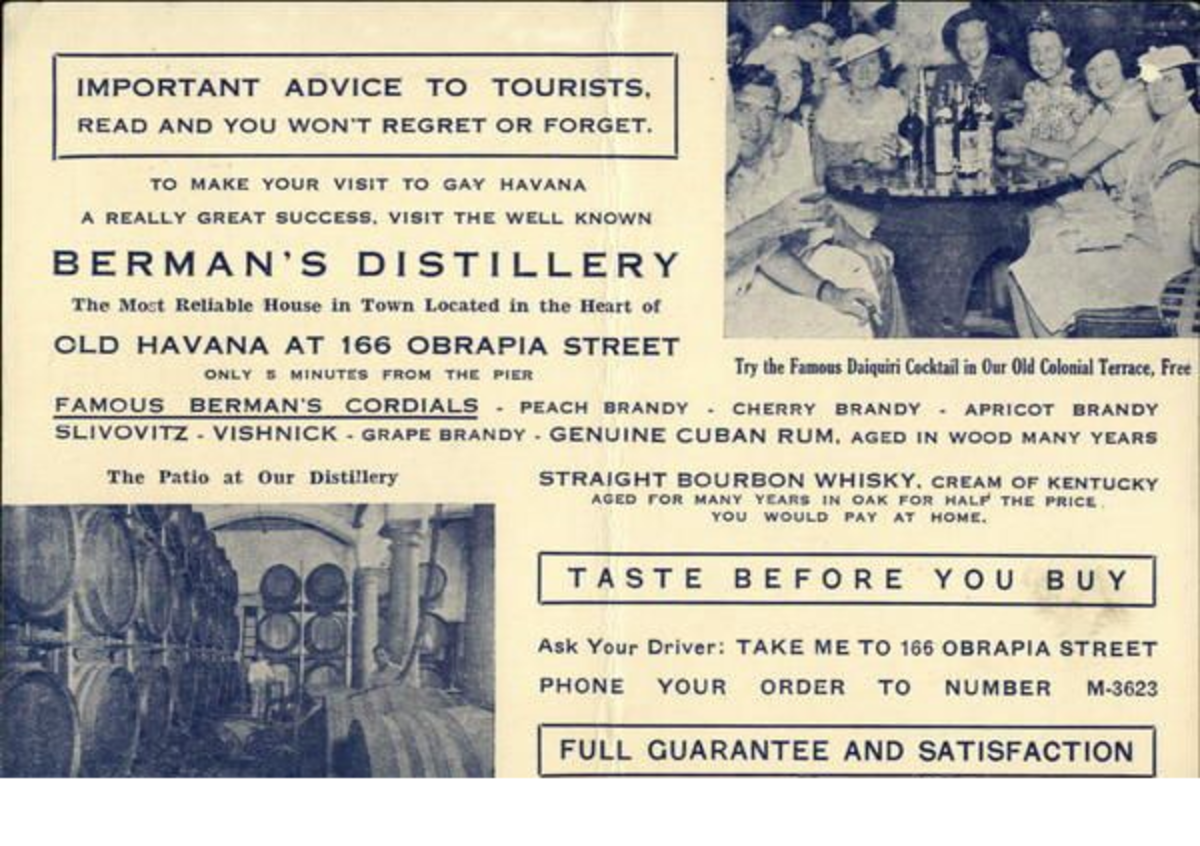The image is an old black-and-white document, possibly an article or a notice, resembling a yellowed newspaper clipping with dark blue text. The top left features a rectangular box stating: "Important advice to tourists, read and you won't regret or forget." Outside the box, it reads: "To make your visit to Gay Havana a really great success, visit the well-known Berman's Distillery, the most reliable house in town located in the heart of Old Havana at 166 Obrapia Street, only three minutes from the pier." 

On the top right, there's a black-and-white photograph of a group of women, with a few men in the background, sitting around a wooden table laden with bottles of alcohol. The caption below this picture promotes: "Try the famous daiquiri cocktail in our old colonial terrace, free."

At the bottom left, another black-and-white image depicts barrels, likely indicating storage or a distillery setting, captioned: "The patio at our distillery." 

The document lists various types of brandy available and concludes with the invitation: "Taste before you buy. Ask your driver, take me to 166 Obrapia Street, or phone M-3623. Full guarantee and satisfaction."